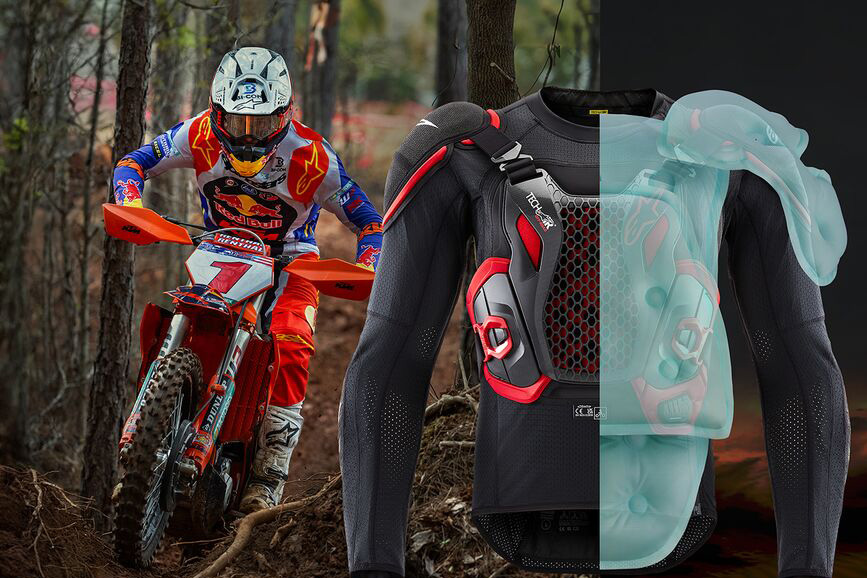The image is a composite advertisement featuring a motorcyclist riding a dirt bike through a forest and a detailed view of protective body armor. On the left side of the image, a professional motorbike rider is navigating a dirt path among dense trees. He is on a red motorcycle with the number "1" on it, wearing a colorful racing suit adorned with Red Bull and other advertisements. His suit includes white boots and a white helmet with a yellow face mask and black and orange chin strap, with the visor reflecting light.

The right side of the image showcases a close-up of the protective armor designed for motorcyclists. This suit features a black and red design with metal mesh covering the chest, a black mesh over the arms and stomach, along with shoulder pads and chest plates for enhanced protection. It also has a transparent section that reveals the internal padding, emphasizing the hard plastic material intended to cushion and protect sensitive areas during a crash. The image effectively highlights the rugged forest terrain the rider is navigating and the critical safety features of the body armor being advertised.